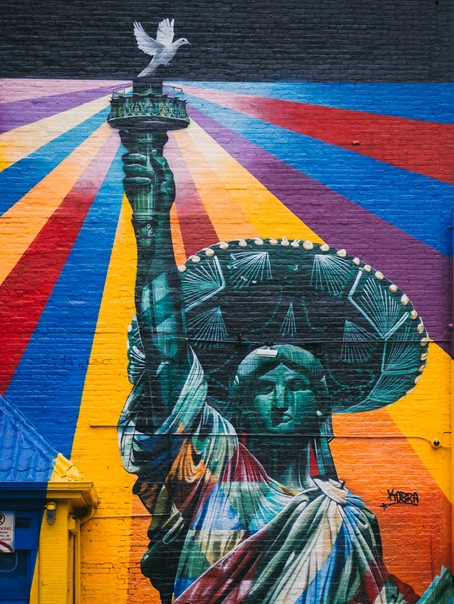The image portrays a vibrant graffiti of the Statue of Liberty on the side of a building. The Statue is whimsically adorned in a colorful, tie-dyed toga-like gown showcasing shades of pink, blue, purple, and white. Positioned on her head is a striking sombrero with intricate shell designs in black, blue, and white hues. Perched atop the torch she holds high is a white dove, symbolizing peace.

The backdrop is a dynamic array of vivid, radiating streaks of light in blue, red, purple, yellow, orange, and pink, converging towards a central point, creating an effect similar to searchlights beaming down from above. Over her left shoulder, a brick section displays the word "COBRA" in bold capital letters marked with a little star. Adjacent to the image, there is an outcropping resembling a door and a sign, possibly indicating "No Parking," though it remains partially obscured.